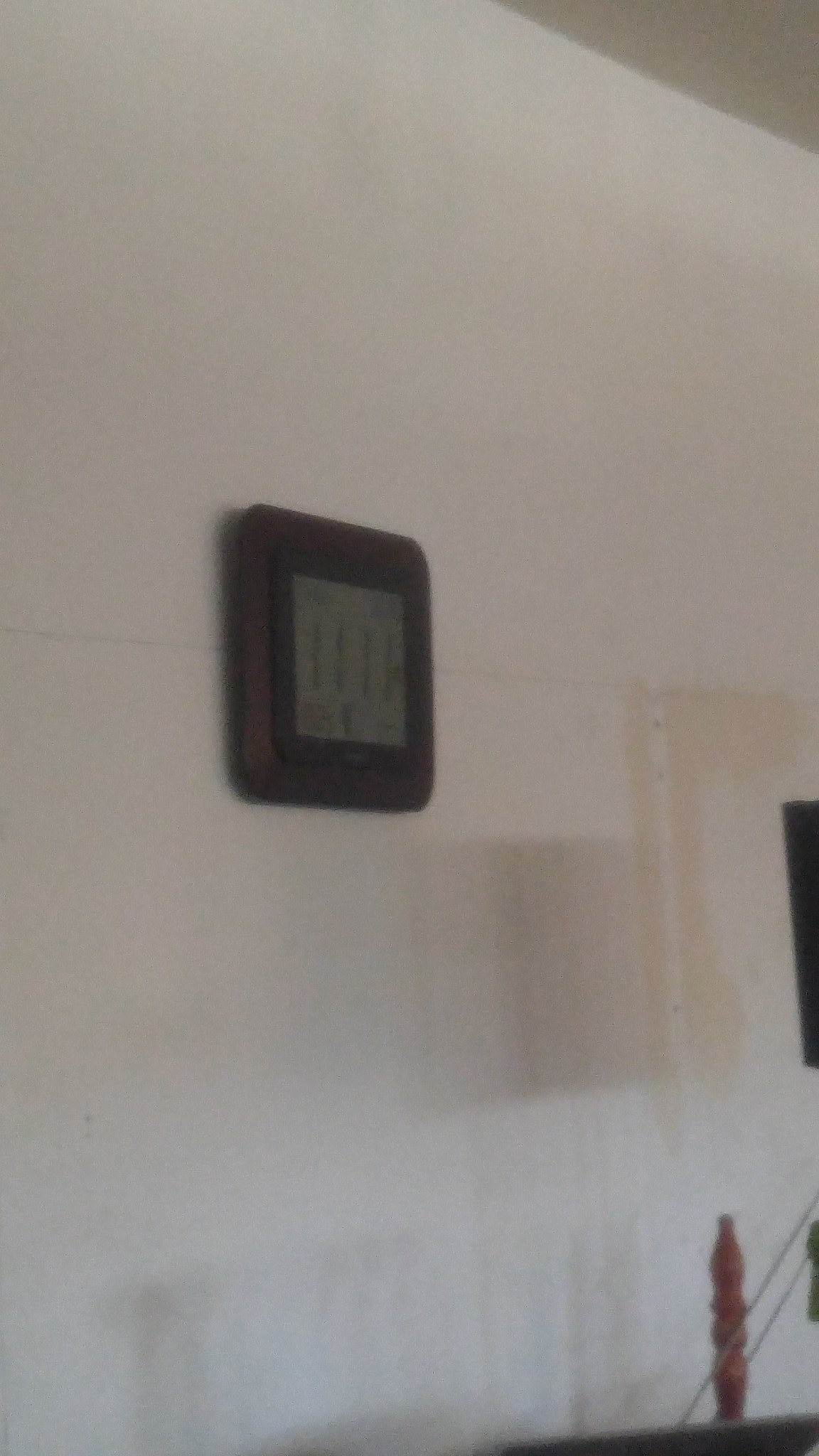A digital wall clock, displaying the time as 11:11, is mounted on a white, shadowy wall. The clock, characterized by its rounded corners and dark gray color, features a plain greenish-gray digital screen that prominently shows only the time. Despite its likely additional functions such as displaying the date and temperature, these details are obscured in the image. The photograph is notably low in quality, appearing very grainy and slightly blurred. The dim room is poorly lit, creating numerous shadows across the wall. Limited light from a window subtly illuminates part of the scene, though it fails to significantly brighten it. Shadows cast by a lamp and possibly a chair or another piece of furniture are visible, along with glimpses of the lamp's shade and base. Beyond these elements, the scene is stark and unembellished.